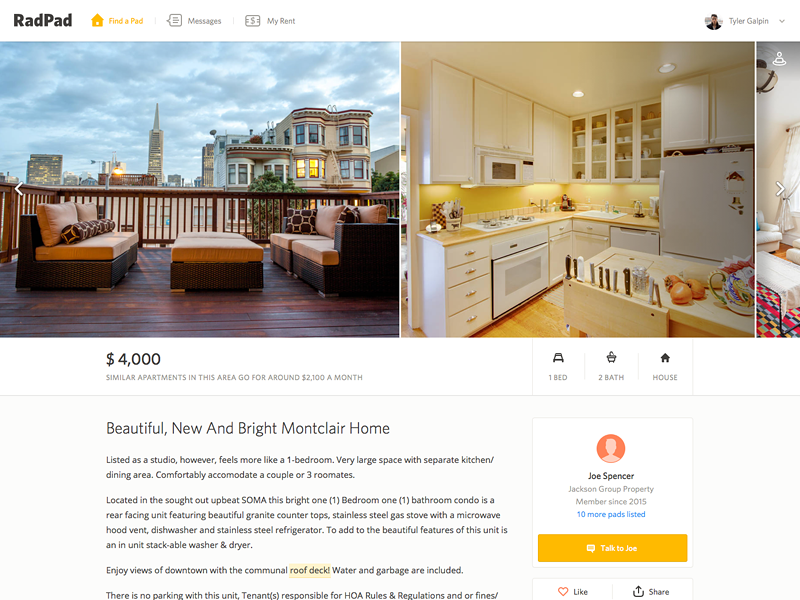The image displays a rental listing from RADPAD, showcasing a luxury apartment in San Francisco. On the left side of the image, there is a photo of a rooftop area that appears to be located in the SoMa (South of Market) district, known for its vibrant atmosphere. 

The right side of the image shows a modern, fully-equipped kitchen featuring beautiful granite countertops, a stainless steel gas stove with a microwave, a hood vent, a dishwasher, and a stainless steel refrigerator. There's also an in-unit stackable washer and dryer for added convenience.

The listing details mention that this residence is a bright one-bedroom, one-bathroom condo, but is labeled as a studio. Despite this, it boasts a substantial living space with separate kitchen and dining areas, making it suitable for a couple or even three roommates. 

The unit is priced at $4,000 per month, significantly higher than the average $2,100 per month for similar apartments in the area. This Montclair home is described as beautiful, new, and bright, with plenty of space to comfortably accommodate its residents.